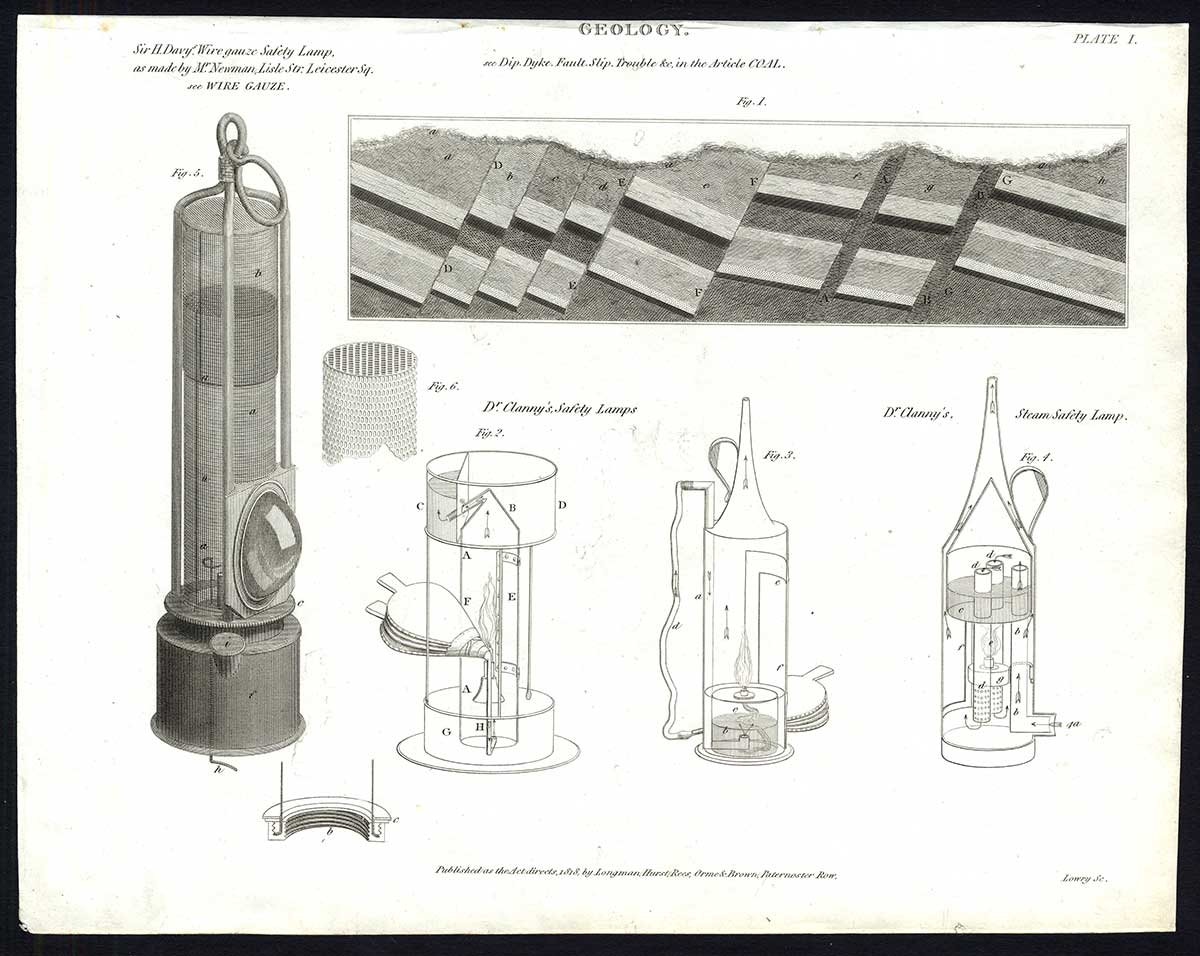This detailed drawing, resembling an old blueprint or instructional scroll, is titled "Geology" at the top and features a thick black frame around its stained white background. In the top right corner, it is labeled "PLATE 1." The upper left corner in cursive reads "Sir H. Davy Wire Gauze Safety Lamp as made by M. Newman, Leicester Square." Below this, the diagram depicts a tall, cylindrical object, possibly the safety lamp itself.

The image also includes a series of labeled components arranged across the center, identified by letters A through G and figures 2, 3, and 4. Adjacent to these components, on the right, there are additional illustrations and labels indicating how the parts interconnect. A rectangular inset at the top shows overlapping square plates, each associated with specific letters, indicative of geological strata or mechanical components.

Partially legible text seems to describe geological features such as "Deep Dyke," "Fault," and "Slip Trouble." Though some small text remains unclear, it appears to detail geological survey elements alongside the mechanical diagrams of what might be Clanny or Davy safety lamps, crucial tools in geology and early mining.